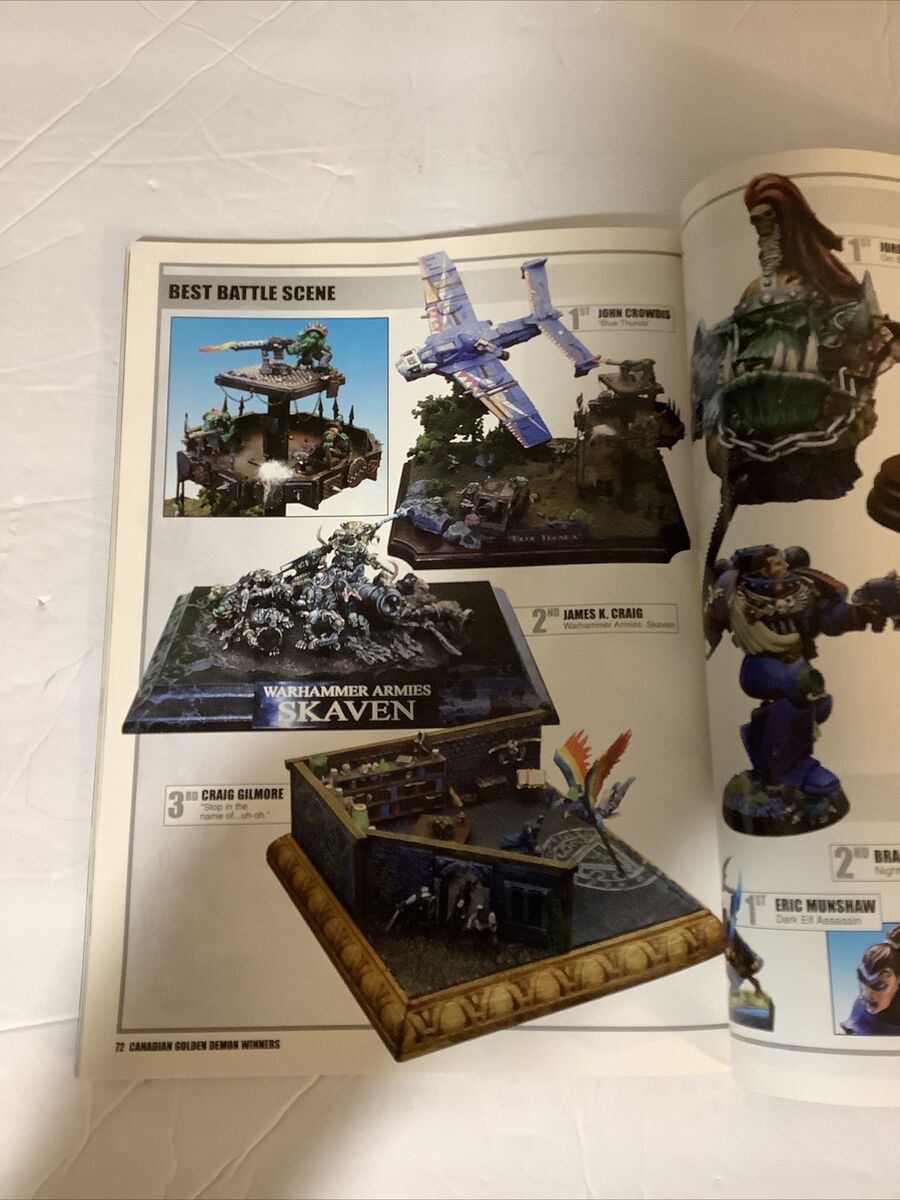This image features a close-up of an interior page from a magazine set against a beige-colored background. The photograph focuses on the left page, which prominently showcases battle scenes with highly detailed figurines and environments. At the top left-hand corner of the page, "Best Battle Scene" is highlighted in black letters against a gray background. Below this heading, there are several illustrations: the first depicts an airplane being shot down by military guns and cannons; the second is titled "Warhammer Armies: Skaven" by James K. Craig, featuring intricate designs of the Skaven faction; the third image is captioned "Craig Gilmore: Stop in the Name of Uh-Oh," showing what appears to be a piece of wooden furniture, possibly integrated into a battle diorama. The right-hand side of the image also includes additional pictures or diagrams, further enriching the visual content of the magazine.